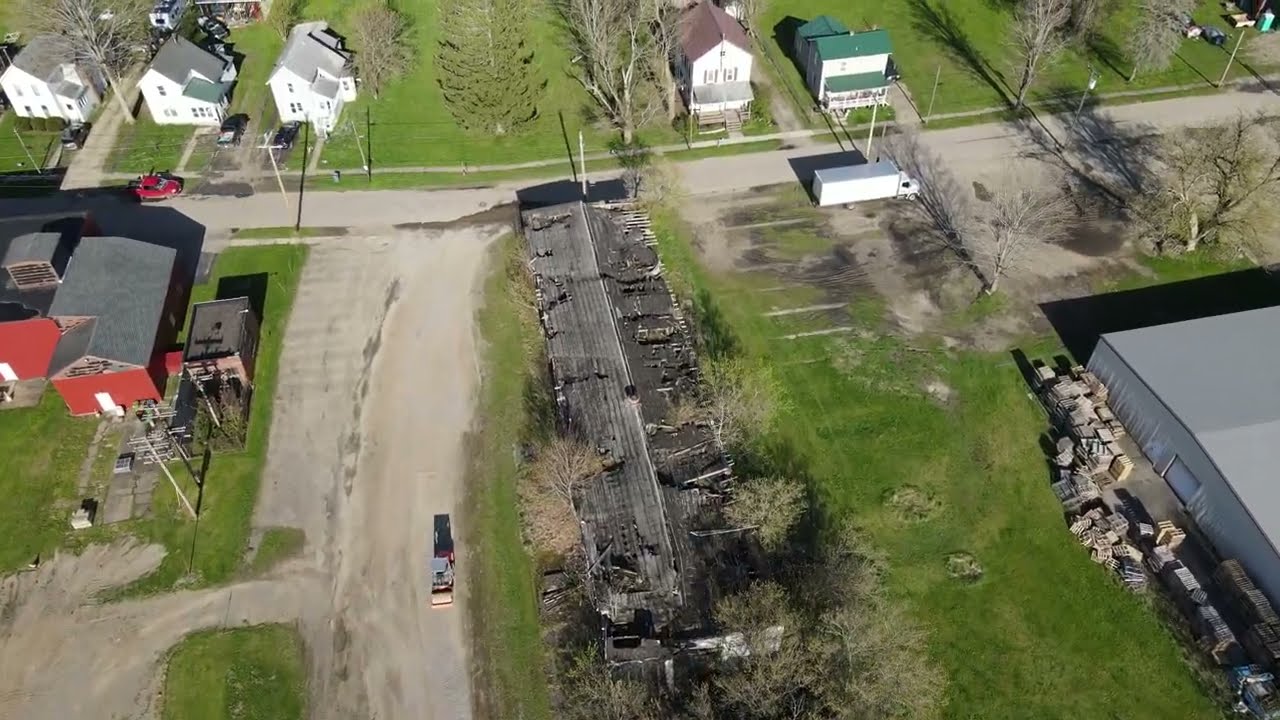This detailed aerial photograph captures a horizontally aligned rectangular image of a rural residential area. At the top of the image, a row of tall, two-story farmhouses with varied roof shapes—predominantly hipped and A-line—in white, gray, and some with brown and green roofs line a road that stretches from left to right. In the middle of the scene, a white semi-truck is parked along the road, which intersects with less paved, perpendicular streets. A red barn with a gray roof stands out on the middle left, accompanied by a vehicle on a sand-colored driveway. Further to the left, there is a black-roofed structure with red buildings amidst patches of green grass. In contrast, the right side of the image features a green grassy field and a gray warehouse with stacked pallets situated at the lower right corner. Scattered throughout the area are bare-branched trees devoid of leaves, accentuating the rural and slightly worn character of the landscape. The overall setting is an outdoor daytime shot, offering a panoramic view of a quaint farm area.